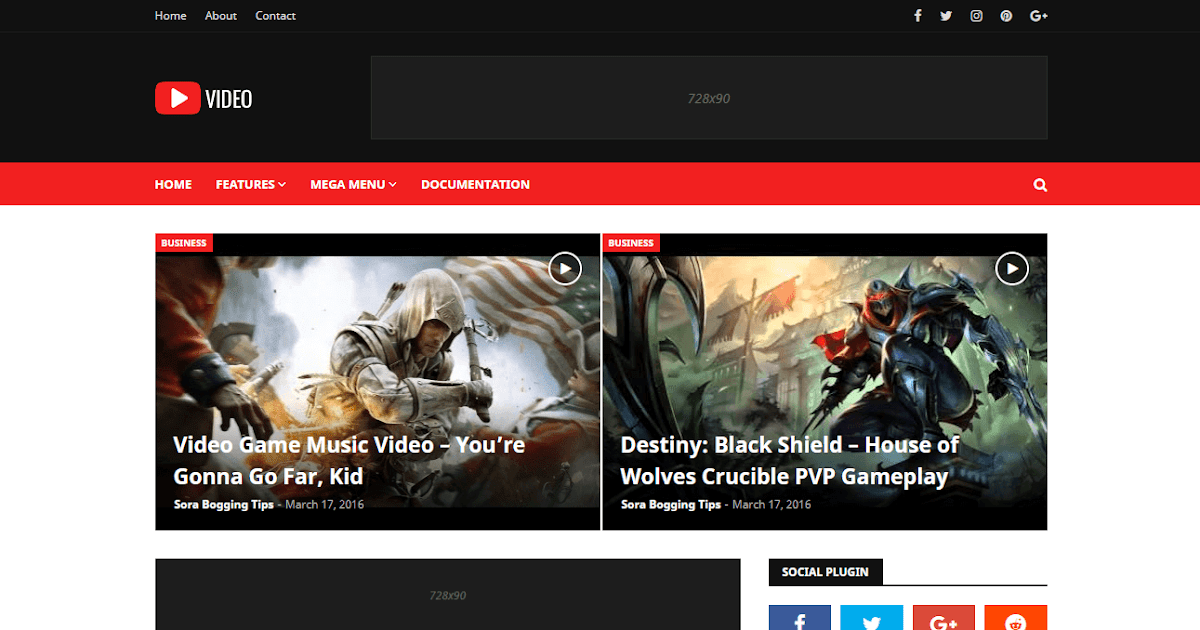The image depicts a webpage designed to resemble YouTube, distinguished by a red rectangle adorned with a white play button icon and the word "Video" in white font next to it. The top section of the page features a black background, with navigation options placed on the edges: "Home," "About," and "Contact" on the left, and icons for "Facebook," "Twitter," "Instagram," and "Google+" on the right.

Below this, on the left side, the YouTube icon along with the word "Video" is repeated, and the center of this section includes the text "27728X90." Underneath, there is a red strip that runs across the webpage. Embedded in this strip are various navigation links presented in red and white font: "Home," "Features" with a dropdown menu, "Mega Menu" with another dropdown, and "Documentation." On the right end of this red strip, there is a search icon.

Further down the page, there are two prominent images positioned side by side. Each image has a red rectangle in the upper left corner with the word "Business" inscribed in white. The left image is titled "Video Game Music Video - You're Gonna Go Far, Kid," while the right image is labeled "Destiny - Black Shield - House of Wolves - Crucible PVP Gameplay."

The lower portion of the page features another black bar containing the text "728X90" on the left and a "Social Plugin" section on the right, which includes icons for "Facebook," "Twitter," "Google+," and "Reddit."